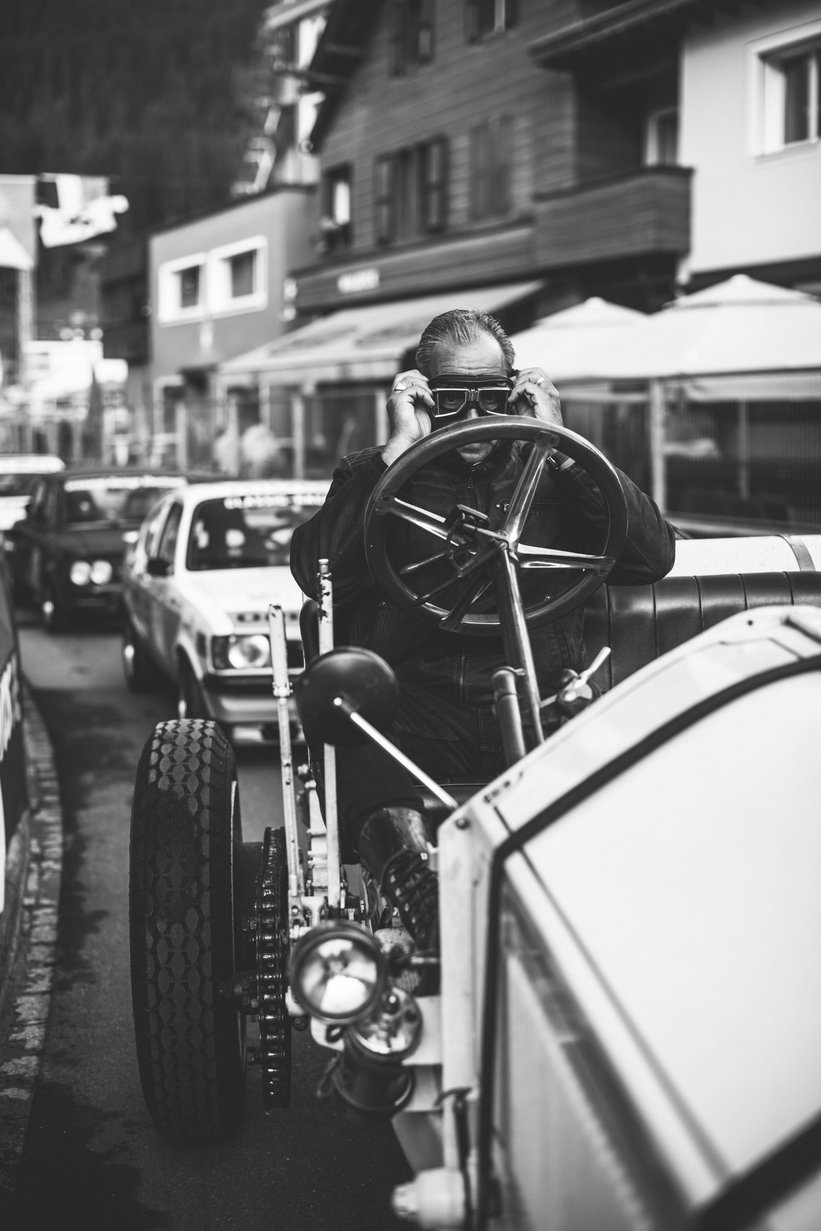In this detailed black-and-white photograph, a man with slicked-back hair is captured in a vintage scene. He is seated in an open-top roadster, which bears a resemblance to an old Indy car or go-kart. The man is in the process of adjusting his goggles, his hands lifted to his face. The vehicle is a convertible with a minimalist design, featuring a prominent steering wheel that juts out from a long, black tube-like pole. Visible on the left side of the car are large headlights, a single wheel, and what appears to be black leather seats.

Surrounding the primary subject are several other older vehicles, indicative of the photo's historical context, possibly the 1970s. These vehicles are lined up on an asphalt road, accentuating the vintage ambiance. The background offers a blurred glimpse of a townscape, which includes multiple buildings that resemble housing units or possibly a shopping area. Some structures appear to be up to three stories high with a fence in front, adding to the urban setting. Additionally, a sidewalk is discernible on the very left edge of the photograph.

Overall, the main focus rests on the intriguing juxtaposition of the man in his unique roadster against the backdrop of a bustling, yet blurred, town.